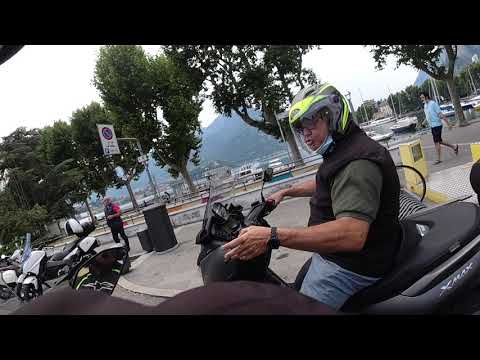In this clear daytime image, we see a man centrally positioned, riding a moped branded X-Max, in the lower right corner of the frame. He is wearing an olive green short-sleeved shirt with a black vest, and a yellow and black helmet with a clear face shield down, revealing his glasses and a COVID-19 mask on his chin. He appears to be pointing towards the left side of the image while speaking to someone off-camera.

The setting is outdoors, possibly in an Asian country, evident from the non-U.S. traffic sign visible in the background. The ground is paved with concrete or asphalt, and a few other mopeds are parked nearby. In the background, a couple of people are walking on the sidewalk next to some trees and garbage cans.

Further in the distance, there are tall, hazy mountains under an overcast sky with minimal clouds, giving the scene a bright but slightly diffused natural light. The image also captures boats docked in a harbor, suggesting proximity to a body of water. The primary colors in the scene include black, brown, gray, white, light green, tan, red, and light blue.